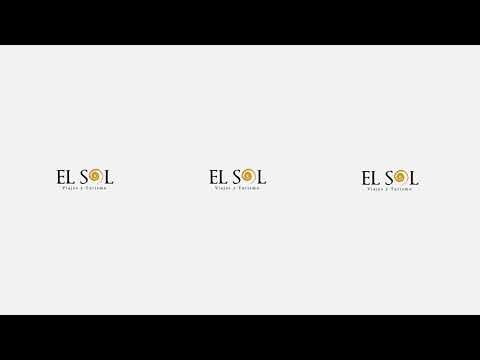The image features a simple, repetitive design framed by thick black horizontal bars at the top and bottom. The central section of the image has a light gray background and prominently displays the business logo "El Sol" three times, evenly spaced from left to right. Each "El Sol" logo is rendered in black text, with the "O" replaced by a distinctive yellow swirl resembling a sun. Directly beneath each "El Sol" is a line of small, unreadable black text that becomes indiscernible upon closer inspection. The overall composition emphasizes the repeated branding against the neutral backdrop, creating a clean and consistent visual pattern.